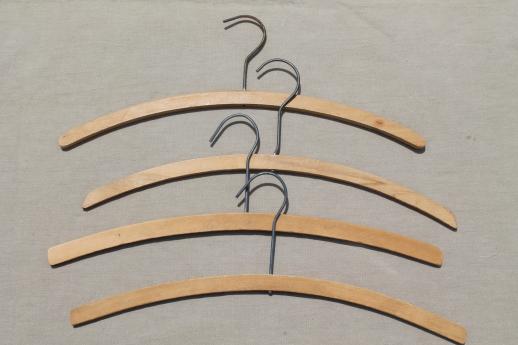The photograph features four vintage wooden hangers with a light golden hue, each equipped with a thin, dull silver metal hook. The hangers, characterized by their gently curved wooden bars, appear aged and reminiscent of those found in a grandmother's closet. They are arranged in a staggered vertical line, with each hook curving to the left. The hangers lie on a dull white or light gray background, creating subtle shadows that give the illusion of double hooks. The arrangement alternates from left to right, enhancing the composition's intriguing simplicity.